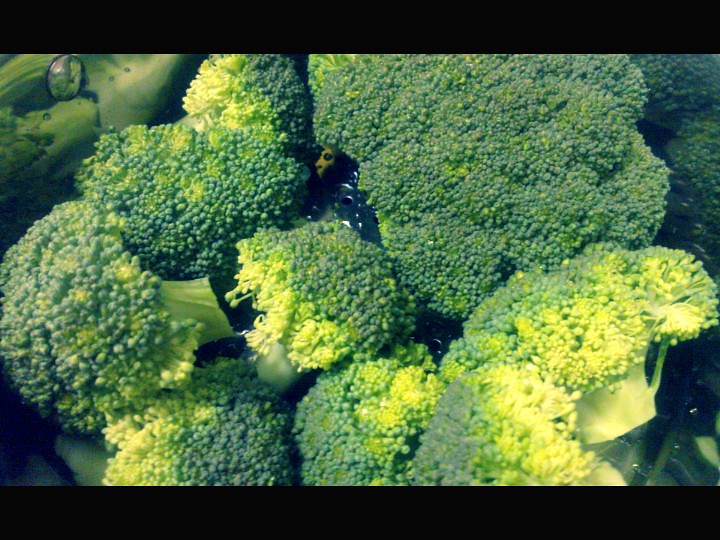This close-up image features a tightly cropped bunch of broccoli heads, roughly eight in total, with the majority being small to medium in size and one particularly larger head. The broccoli heads, neatly cut with short stems just above the florets, are predominantly a deep green color with some edges tinged in yellow and lighter green hues. The background reveals hints of celery stalks, suggesting the setting might be a market or a preparation area. The broccoli appears dry yet edible, arranged on a black surface with visible holes, and black bars frame the top and bottom of the image. The overall composition emphasizes the freshness and detail of the broccoli heads, highlighting their natural texture and color variations.